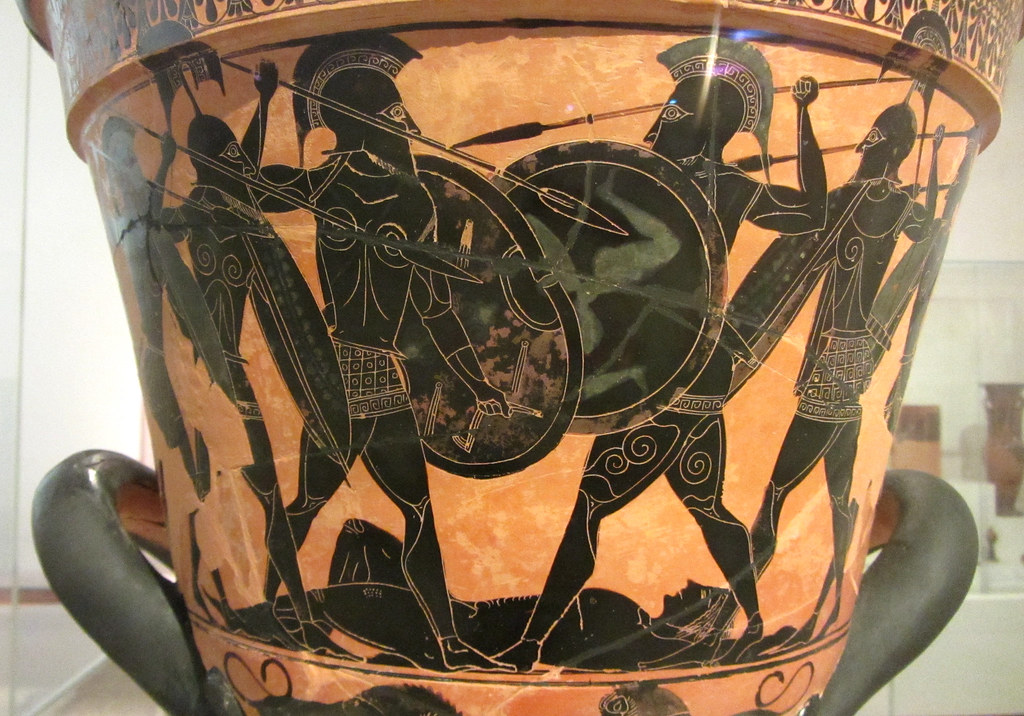This photograph depicts a close-up of an ancient ceramic vase with finely detailed etchings and depictions of Greek or Spartan soldiers. The vase, which appears to be a museum artifact due to its aged and imperfect surface, is primarily orange with black-painted designs. These designs, rendered in a somewhat abstract style, feature soldiers engaged in combat, adorned with detailed armor, crested helmets, and round shields while wielding spears. One soldier is shown lying on the ground, suggesting a narrative of battle and defeat. The vase includes two black handles towards its lower portion, enhancing its practical use while adding to its ornate design. Despite the image cutting off at the top and bottom, the intricate spiral etchings depicting the muscles and armor are clearly visible.